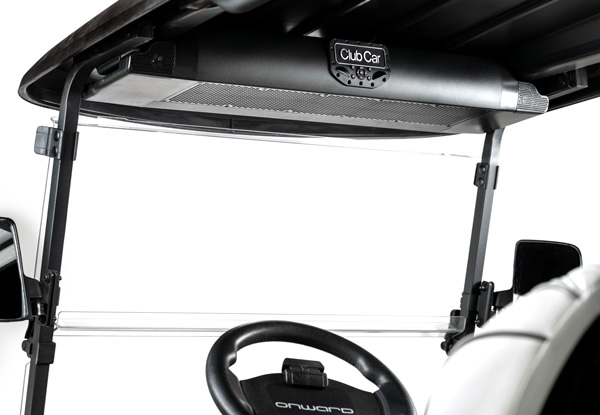This black and white photograph captures the front interior of an older model golf cart against a white background. The image is dominated by a black roof with a logo displaying "Club Car" in white letters at the top center. Black metal poles descend from the roof on either side, supporting a transparent windshield positioned in front of the steering wheel. The steering wheel, also black and emblazoned with some illegible white text where the horn would be, is partially visible. On both the left and right sides of the cart, black side-view mirrors are mounted, although they are slightly cut off in the frame. The visible part of the seat beneath the steering wheel shows a white material with some folded detailing. The focus of the image is clearly on the inside of the cart, which is bathed in consistent white light that emphasizes the contrasting black elements.